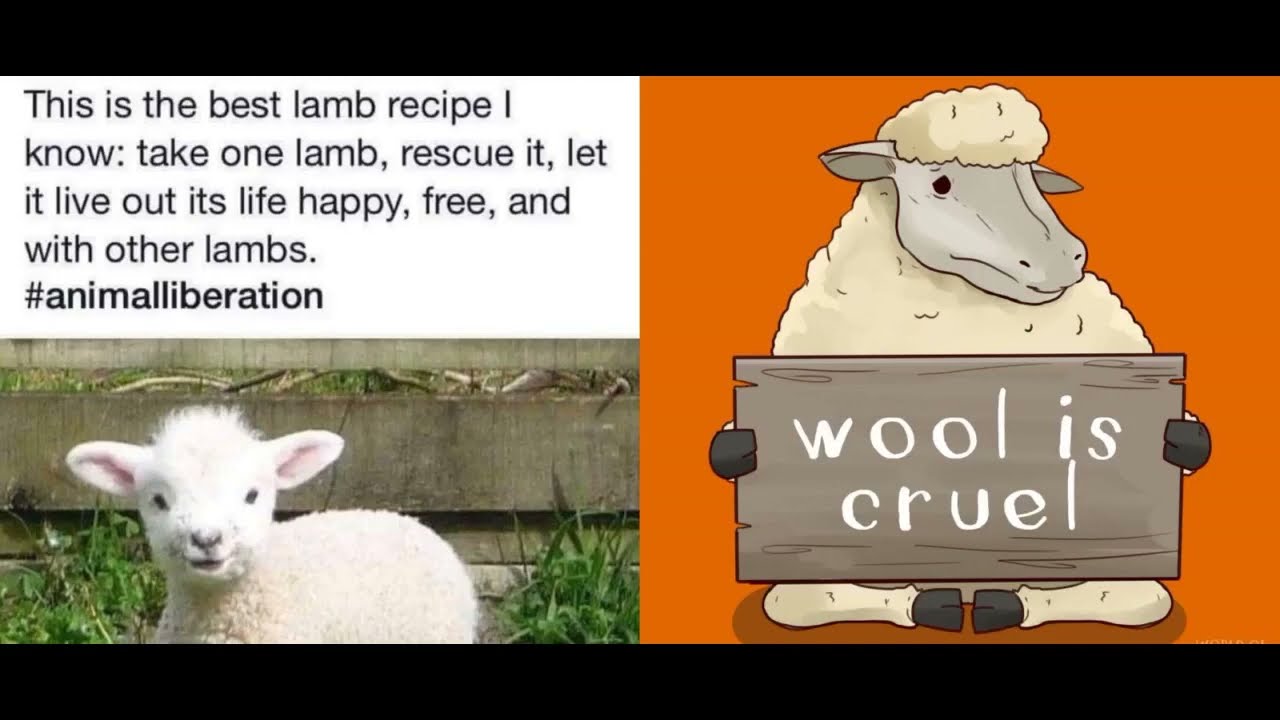The horizontal rectangular image is neatly divided into two main parts. On the right side is a bright orange background featuring a charming cartoon lamb with off-white puffy wool. Sitting cross-legged, the lamb hoists a wooden sign with the handwritten message "Wool is cruel." 

On the left side, the image is split into two sections: a white rectangle at the top and a photograph below it. The white rectangle displays black text that reads: "This is the best lamb recipe I know: Take one lamb, rescue it, let it live out its happy life, free, and with other lambs." Beneath the text is the hashtag "#animalliberation." 

Below the text is a real photograph of a baby lamb standing outside in a grassy area beside a wooden fence, looking adorable as it smiles at the camera. The image, bordered by black strips on the top and bottom, appeals to viewers to consider animal liberation and avoid products derived from lambs.